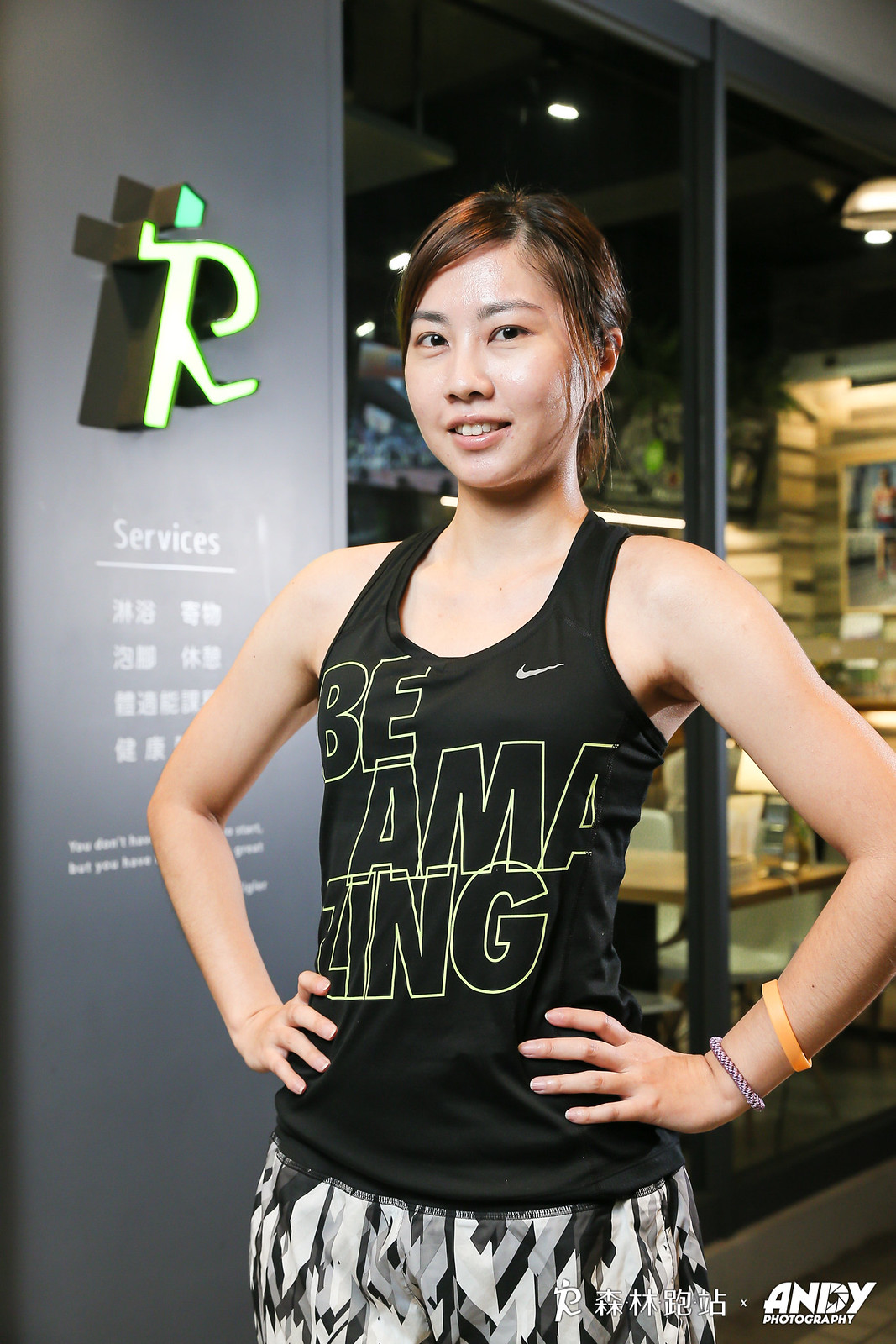This vibrant photograph features a young and pretty Asian girl, confidently smiling into the camera. Standing indoors, the girl strikes a powerful pose with her hands on her hips. Her sleek brown hair is pulled back in a ponytail, with a small lock of hair elegantly hanging by her ear. She is dressed in a black Nike tank top with the emblazoned motivational text "B-Amazing," separated into "B-A-M-A" and "Z-I-N-G" on the following line. Complementing her athletic outfit, she wears black and white patterned running shorts. Her right wrist is adorned with a purple braided band and an orange bracelet.

The background captures an atmosphere that resembles a gym or training facility, with blurred images suggesting tables or equipment and two windows framing the scene. Prominently, there is an illuminated signage that appears to be an italicized letter 'R' or possibly a running figure, followed by the word "services" and several unreadable Chinese symbols. The photograph is credited to Andy Photography, indicating his name at the bottom of the image.